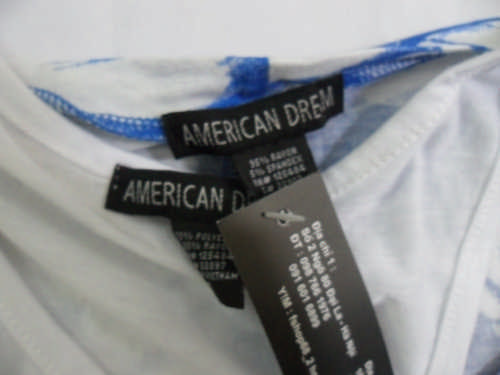This image showcases two pairs of bikini-style women's underwear, prominently displayed. Both pairs are predominantly white with a distinct blue marking situated on the back. The waistband of each pair features the phrase "American Dream." Additionally, there are two tags attached: one clearly reads "American Dream," while the other, albeit slightly blurred, specifies the fabric composition as approximately 95% of another material and 5% spandex.